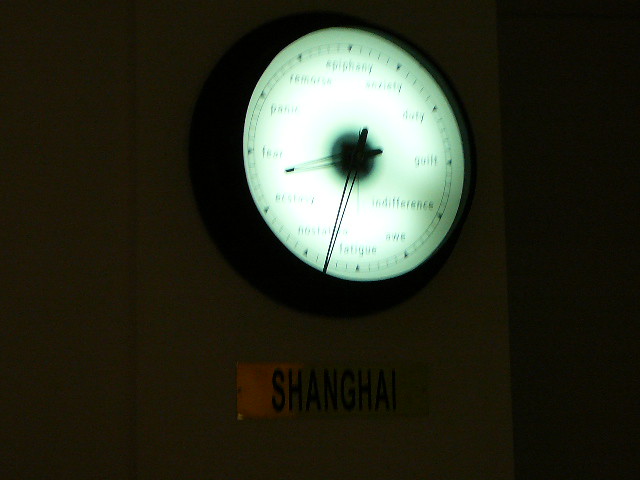The photograph depicts a blurry image of a clock, centrally positioned in the upper half of a rectangular frame. The background is predominantly dark except for an amber hue in the lower left region, where a square object is slightly offset. The clock itself is circular and illuminated with a cool greenish-white light. It features distinctive black arrows marking the hour sections, accompanied by lines between them. Instead of numbers, the clock displays words such as "epiphany," "anxiety," "duty," "guilt," "indifference," "awe," "fatigue," "fear," "panic," and "remorse." The clock hands are triangular and open, with one being longer than the other. The center of the clock is dark, adding to its enigmatic appearance. At the bottom of the clock, there is a metallic sign with the word "Shanghai."